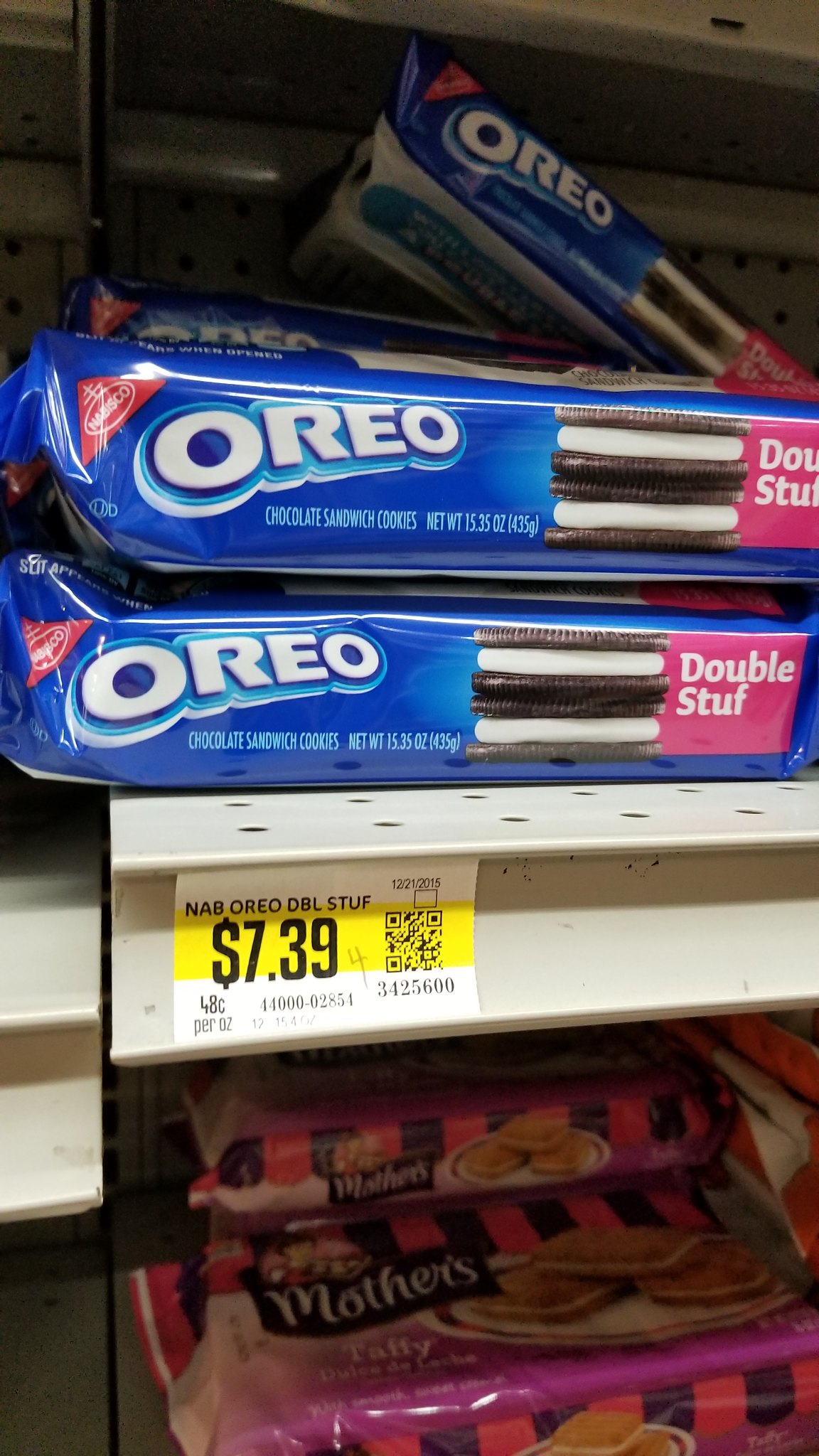The photograph captures a grocery store shelf laden with Oreo Double Stuff cookies and Mother's Cookies. Central to the image is a light metal shelf perforated with holes, prominently displaying three bright blue Nabisco Oreo Double Stuff packages. Two of the Oreo packages are neatly stacked, while the third leans awkwardly at an angle in the background. The distinctive Oreo packaging features the classic blue color with a red Nabisco triangle in one corner and "Double Stuff" highlighted in pink on the other side along with an image of the cookies. A white and yellow price label beneath the Oreos reads "NAB Oreo DBL Stuff $7.39" and includes a QR code. Below this shelf, though slightly out of focus and in a darker area of the photo, there are neatly arranged packages of Mother's Cookies, recognizable by their pink striped packaging. The adjacent shelf is slightly offset, not perfectly aligned with the Oreo shelf, adding a bit of visual asymmetry to the scene.